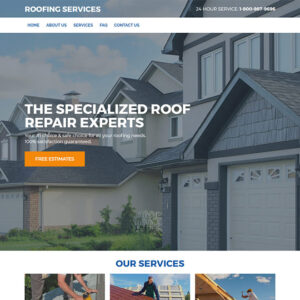The image depicts various aspects of roof services. 

At the very top of the image, a long, narrow rectangular bar features the text "Roof Services" in large white capital letters. Next to that, it states "24-hour service" along with an associated 800 number. The font is slightly blurry, but the essential information stands out. There is also a white background containing a menu with several options in blue capital letters: Home, About Us, Services, FAQ, and Contact Us.

Below this header, there is a large central image showcasing a cluster of two-story houses. The primary house, central in the image, is a grayish color and displays a visible roof, a couple of second-floor bedroom windows, and a two-car garage. To its right is a beige-colored house, where the side of the house, part of the garage, and a fraction of the second floor are visible. On the far right, another house partially in view exhibits a brick color, with a small portion of the second floor visible, hinting at a well-maintained neighborhood.

Overlaying this image, a caption reads "The Specialized Roof Repair Experts." There is smaller text below, which is illegible, but an orange box stands out with the text "Free Estimates," indicating it is clickable.

At the bottom portion of the image, a plain white background features the text "Our Services" in blue capital letters. Below this text are three images depicting various roofing activities. The first image shows an individual actively working on a roof. The second image also features someone working on a roof, but this time the cloudy sky is more prominent, and a man is positioned to the side with a building visible behind him. The final image displays a man on a ladder near a roof, not interacting with it directly, but closely observing the area.